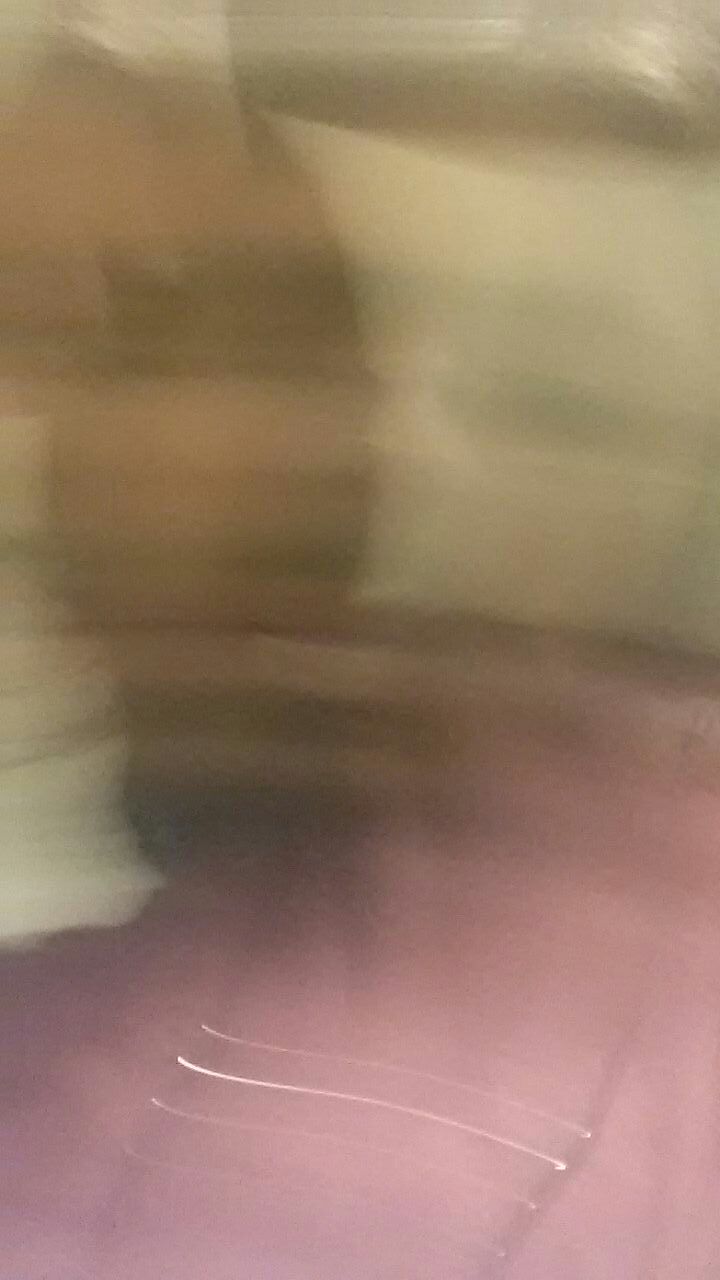This photograph is heavily characterized by motion blur, obscuring the clarity of the image. The scene is a whirl of colors and textures: the bottom part of the image is dominated by a vibrant pink hue, interspersed with four bands of white light that stretch across the frame in a hazy blur. On the left side, there is a patch of black that suggests the appearance of hair or fur, hinting at the possible presence of an animal. The upper right corner features a gradient of white and gray colors, blending into the rest of the image. Overall, the photograph presents a dynamic smear of colors and lights, creating an abstract, almost impressionistic visual effect.